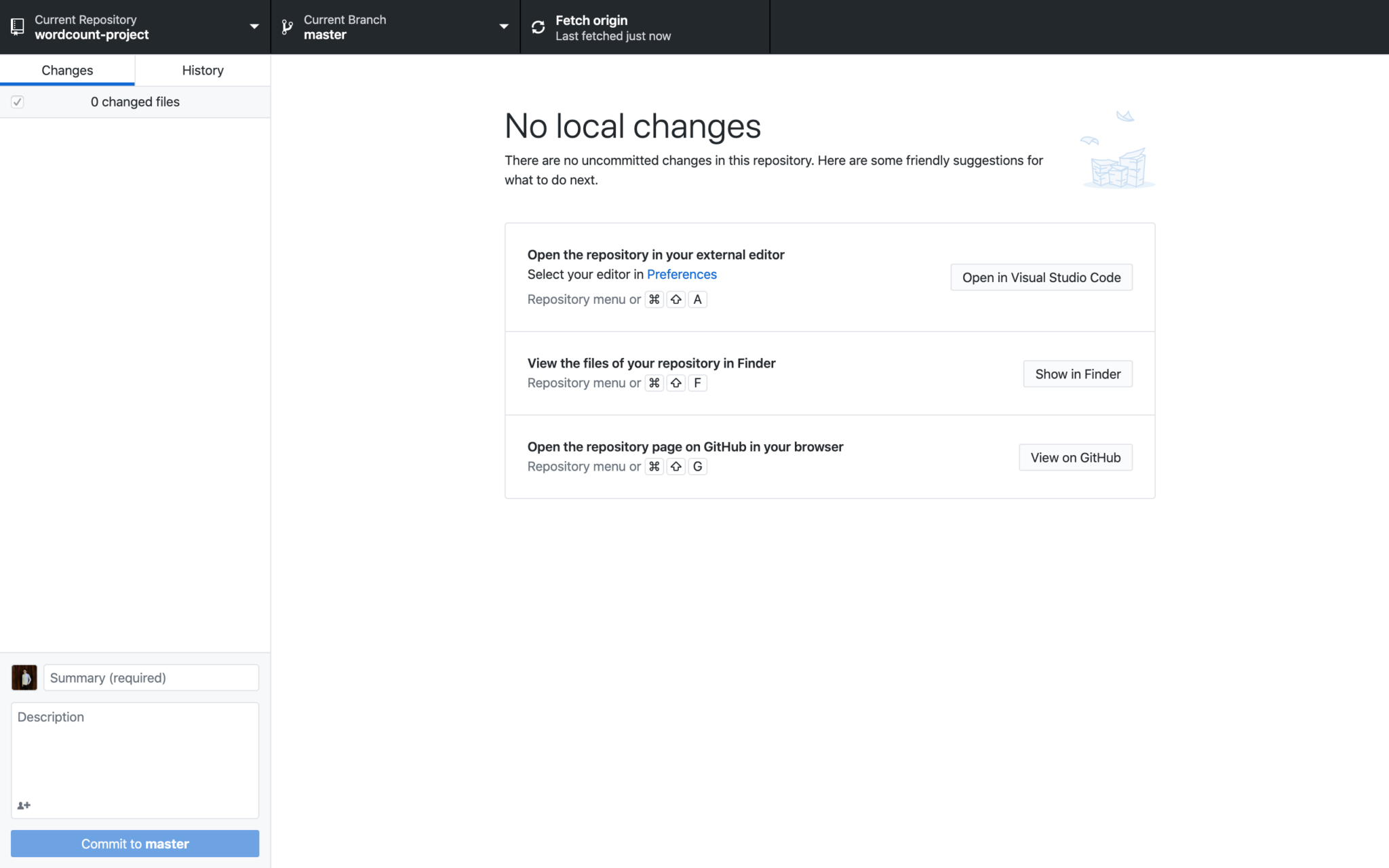This photo captures the interface of a Git management system with multiple detailed elements. At the top of the image is a long black rectangle. To the left within this section, we see the terms "Current Repository" with "Word Count Project" labeled underneath. To the right, it displays "Current Branch" with "master" below it, followed by "Fetch origin" and "Last fetched just now".

On the left side below these labels, there is the word "Changes" underlined in blue, and to its right, the word "History". Beneath these headers, a light-colored rectangle displays "0 changed files". In black text beside it, the message "No local changes" is shown. Underneath, the statement "There are no uncommitted changes in this repository" is written, followed by "Here are some friendly suggestions for what to do next".

The next section includes several actions: First, in black text, "Open the repository in your external editor" is written, followed by the word "Preferences" in blue. The next line within a rectangle reads "Open in Visual Studio Code", and "View the files of your repository in Finder" followed by "Show in folder" to the right.

On the third row, another action is presented: "Open the repository page on GitHub in your browser," with "View on GitHub" written to its right. 

Lastly, in the bottom left corner, the word "Summary (optional)" is labeled, and below it, there's a square for a "Description".